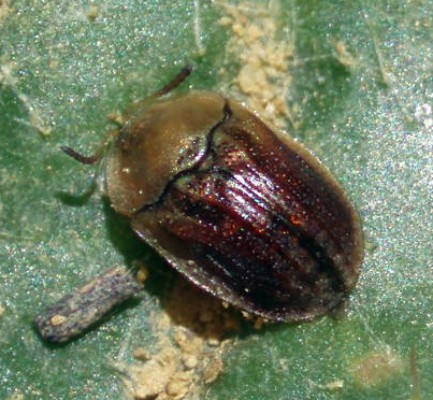This close-up color photograph features a small brown beetle perched on a vibrant green leaf. The beetle, positioned with its head pointing toward the top left corner and its tail toward the bottom right, has an oval-shaped, somewhat reflective shell. The shell's back portion is a darker brown with subtle red and black hues and has distinctive darker red stripes, totaling four, adorned with tiny yellow spots. The beetle's head is lighter, a dark tan or beige color, with a scalloped edge where it meets the darker back. Two brown antennae extend from the front of its head, one straight out to the side and the other crooked upward. The beetle is navigating a green leaf that features a streak of yellow, crusty substance from top to bottom, resembling sand or dirt, and a small brown twig beneath its body. Emphasizing the details, the image appears to have been taken with a flash, as indicated by the white reflections on both the beetle's shell and the leaf. The photograph's style is representational realism, focusing intently on the beetle and the immediate surrounding leaf in a square format.